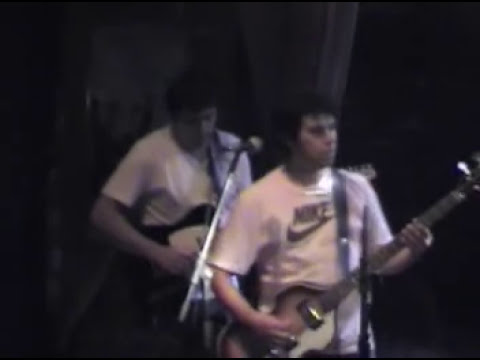In this somewhat out-of-focus and dark picture, we see two men with dark hair, standing one behind the other, engrossed in playing their guitars against a dark brown or black backdrop. Both men are wearing white t-shirts; the man in front sports a Nike t-shirt with the iconic word and swoosh logo, while the man behind him wears a plain white shirt. 

The man in front, positioned slightly to the right, is playing an electric guitar, with his left hand on the neck and his right hand on the strings. A silver microphone stand is off to his right, partially obscuring him. Behind him, the second man, also holding a guitar, which appears to be dark-colored, is looking slightly downwards and has a strap over his shoulder. 

The background features an archway that leads to a completely dark space, with indistinct objects visible beyond the arch. There appear to be shades of a lighter curtain or some light-colored shapes partially visible behind the men, adding a textured aesthetic to the otherwise dim scene.